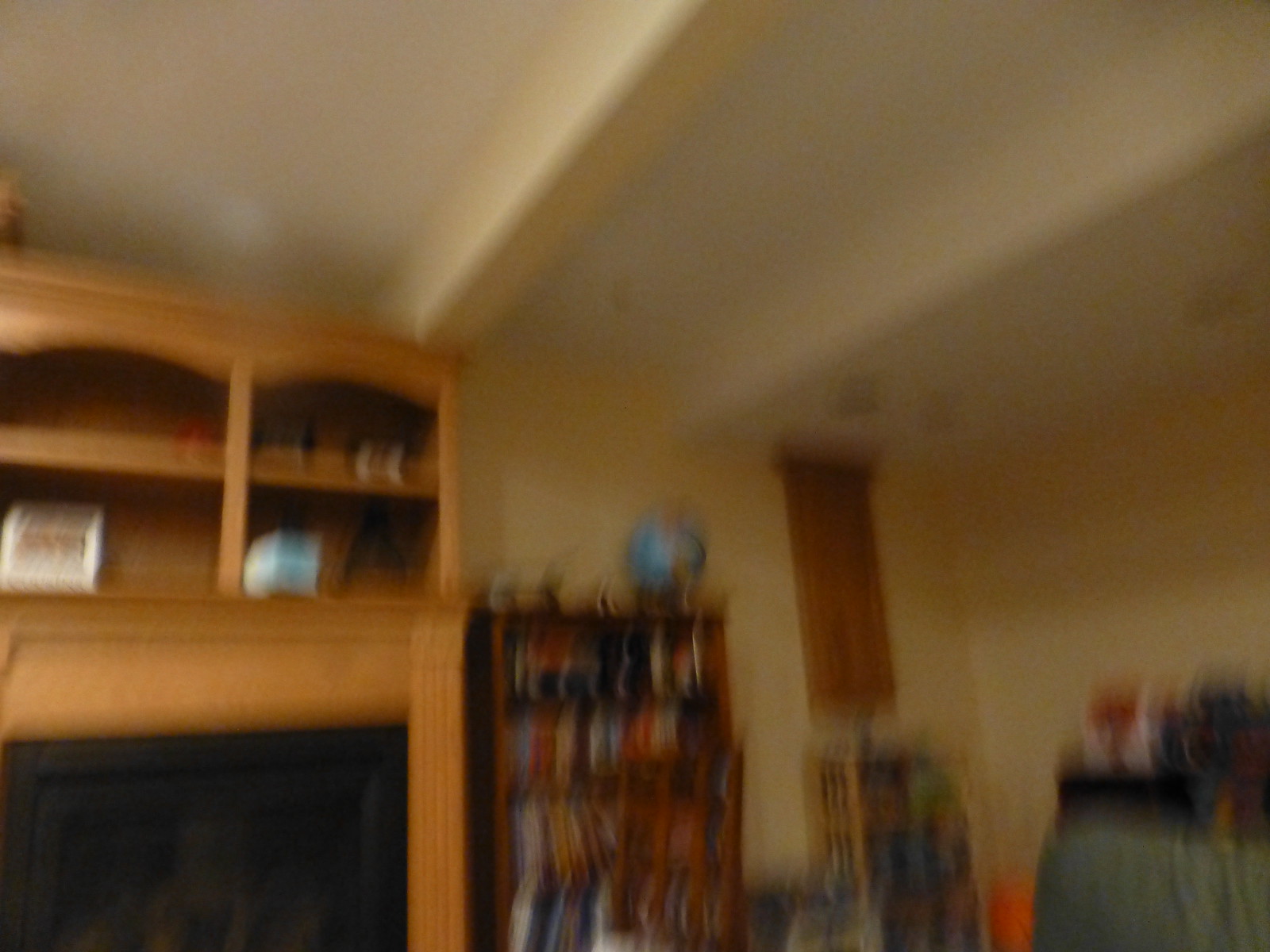This image is a very blurry photograph of a living room in a house, primarily focused on the right corner and ceiling. The ceiling is adorned with white-painted log beams crossing it, and the walls are a tan color. Dominating the right side of the image is a large wooden fireplace mantle that extends up to the ceiling, featuring built-in storage and presentation spaces, including wooden shelves. A black fireplace with a metal front is integrated into the mantle. To the right of this structure, a smaller wooden bookcase stands with a globe perched on top. Against the back wall, there is another bookcase, painted green, and it is accompanied by what appears to be an assortment of other indistinct objects due to the blurriness of the photo. Additionally, there is mention of a hanging red flag between the two bookcases, though it is faint. On the left side of the image, an armoire-like entertainment console crafted from light brown wood houses an old-fashioned square TV from the 90s, with shelving units situated above it.